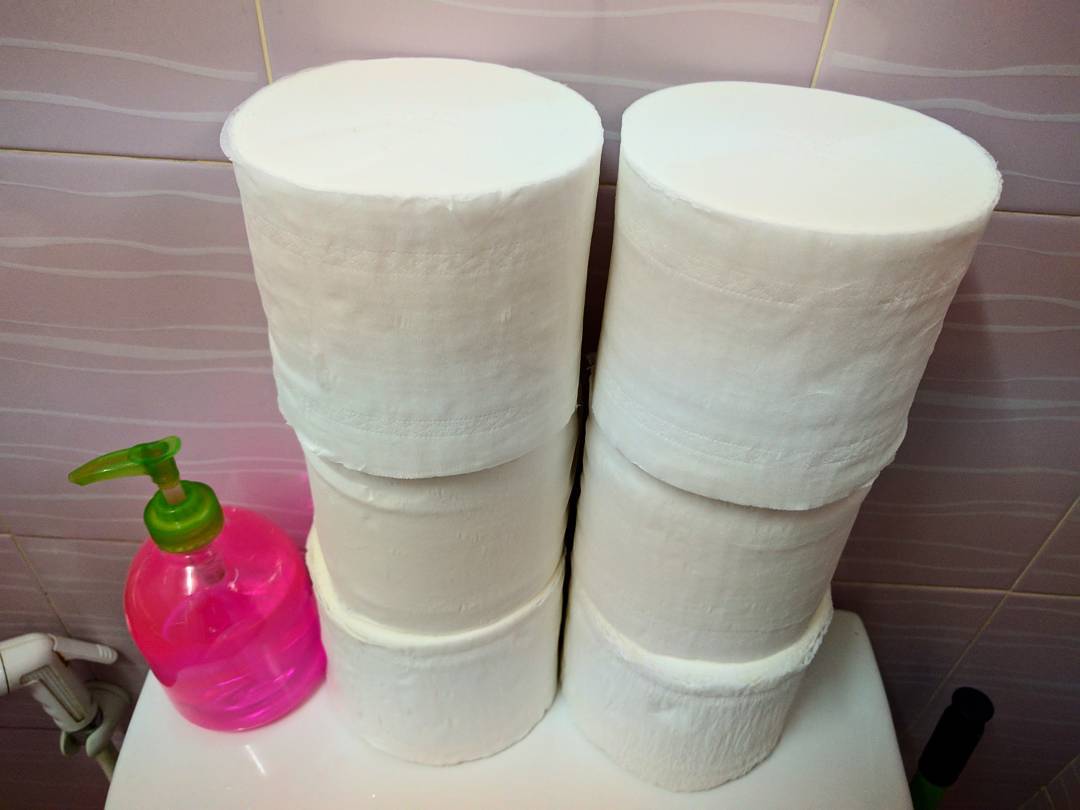The image is a close-up photograph of a white toilet tank with six toilet paper rolls and a pink soap dispenser placed on top. The rolls, each entirely cylindrical without inner tubes, are neatly stacked into two vertical columns of three each. The soap dispenser, bright pink with a clear liquid inside, has a lime green dispensing handle. A white sprayer attached to a wall hook is visible to the left, while a faintly violet, ceramic-tiled wall with cream-colored wavy stripes forms the backdrop. The tiles create an ocean-like effect, adding texture and color to the scene.